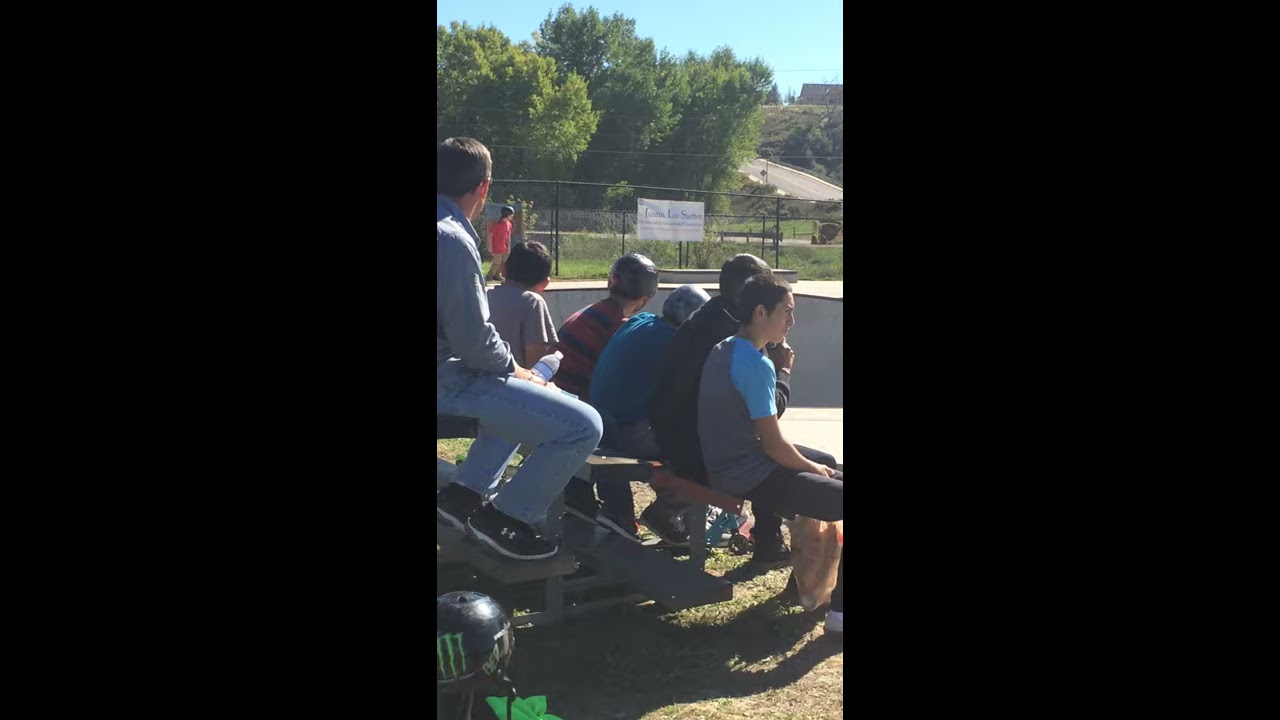The image is divided into three sections, with the first and last sections having a black background. The central section features an outdoor skate park scene with two rows of bleachers set on a grassy area. A total of six men are seated on these bleachers, all appearing to look either slightly ahead or to their left. 

The first row of the bleachers has four men: one in a gray t-shirt, one in a red and blue striped t-shirt, one in a blue t-shirt, and one in a dark jacket. The second row has two men: one wearing a short-sleeve gray and blue t-shirt with shorter pants, and another in a gray sweatshirt, blue jeans, and black tennis shoes.

Behind the bleachers is a mesh wall with an unreadable sign. In the distance, a person wearing a red outfit and helmet is seen near the skate bowl, possibly preparing to skate. The park is surrounded by luscious green trees and enclosed by a fence. Near the foreground, close to the camera, there is a helmet with a monster logo on it. The attention of the seated men is directed leftward, possibly towards an ongoing activity at the skate park.